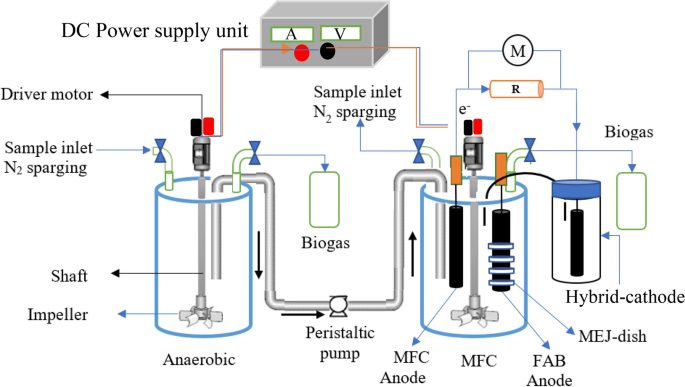The image appears to be an intricate diagram from a science book or technical manual. It features a DC Power Supply Unit labeled in black text at the top left. Adjacent to this label is a gray box with two buttons – one red, marked with the letter 'A,' and one black, marked with the letter 'V.' Below the gray box, there are two cylindrical tubes in the diagram. 

From the red button, lines extend downwards, connecting to a cylinder designated as the "Driver Motor." Nearby labels indicate a "Sample Inlet" and "Sparging." Below this, the shaft is labeled, followed by a component identified as an "Impeller," situated above the term "Anaerobic." 

Proceeding to the right, a pipe connects to a smaller tube labeled "Biogas," continuing downwards to a valve termed a "Peristaltic Pump." This pipe extends further right to another cylinder, which is connected to various labeled tubes. These tubes include "MFC Anode," "MFC," "FAB Anode," and "MEJ dish." 

To the right of this assembly, a sign pointing upwards indicates another "Sample Inlet" and "Sparging." Further elements include a circle marked with an 'M,' a battery symbol with an 'R,' and a cylinder labeled "Hybrid Cathode." The diagram continues on the right-hand side with another label for "Biogas." 

The entire diagram is set against a plain white background, presenting a clear and detailed view of each component and connection within the system.